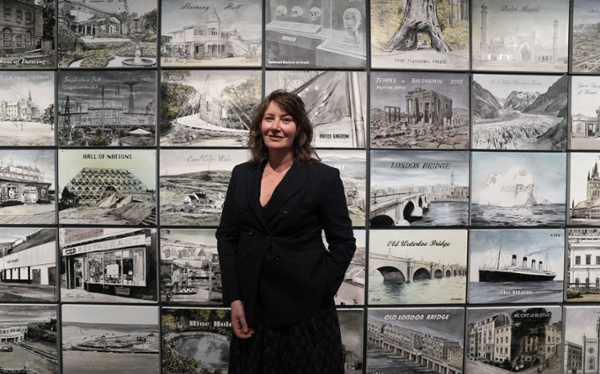In this full-color indoor photograph, a middle-aged Caucasian woman with shoulder-length brown hair stands smiling in front of a wall adorned with numerous black-and-white historical photographs. The photographs, meticulously arranged in squares, feature various subjects including ships, old buildings, bridges, houses, water scenes, and even human skulls towards the top center. The text on these photographs is too small to read. Wearing a blue suit, the woman has one arm gracefully placed behind her back and the other rested beside her. Her attire, which combines elements of both casual and business wear, consists of a v-neck top complemented by a black jacket. The wall of images, rich in historical significance, creates a compelling and intricate backdrop for this portrait.